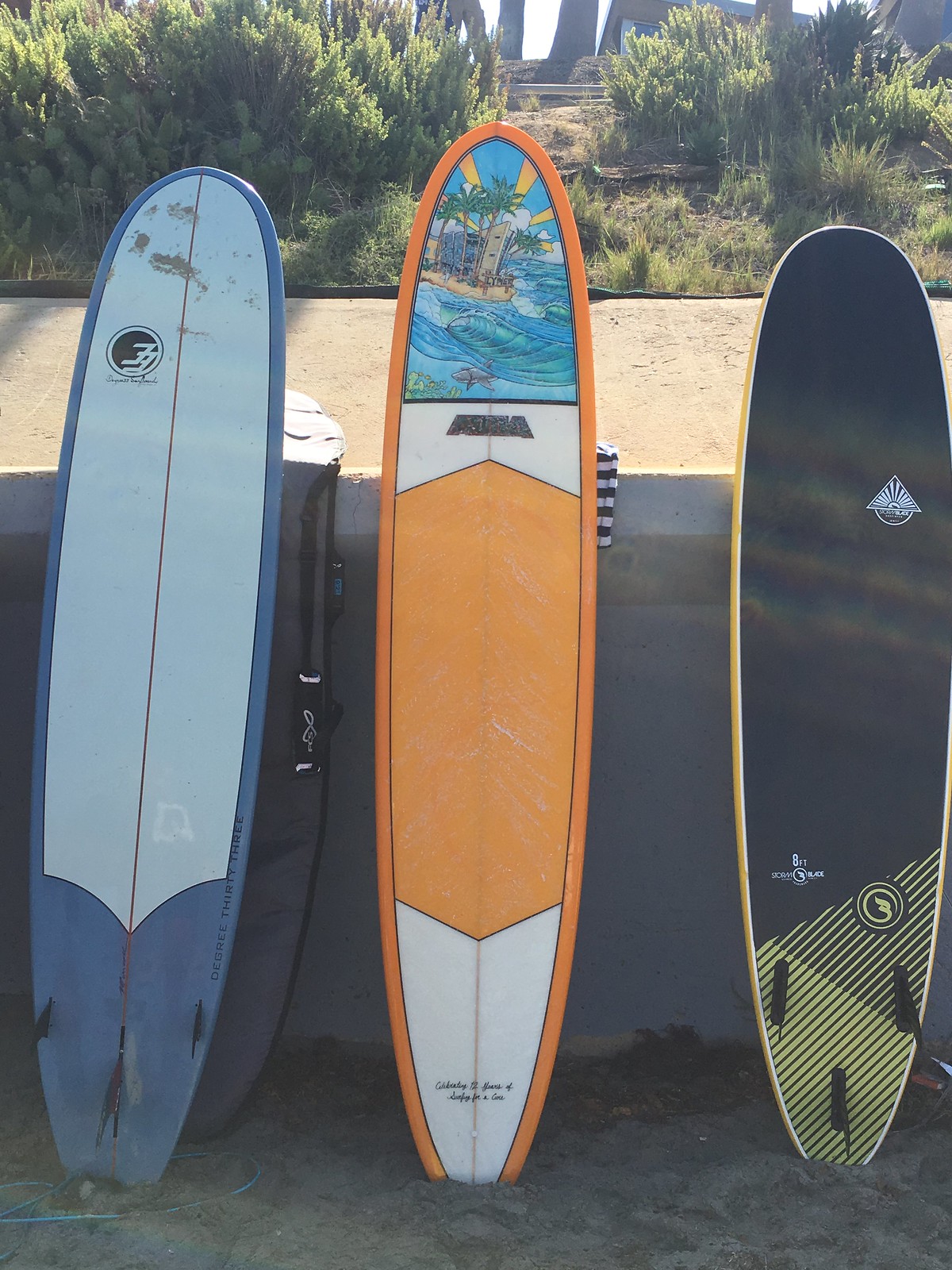This vibrant urban surfer-style image features three surfboards partially embedded in the sand and leaning against a concrete break wall, with a sunlit sidewalk atop the wall. The backdrop includes a scatter of small trees and leafy foliage. 

In the center is an eye-catching orange surfboard adorned with a colorful graphic depicting a seaside scene with water, fish, palm trees, and the sun. To its left stands a dark blue and light blue surfboard bearing a surf brand logo. The rightmost surfboard is predominantly black with striking yellow lines near its base. The image, suitable for sharing on social media platforms like Facebook or Instagram, captures the essence of a laid-back beach day, perfectly complemented by the sunny weather.